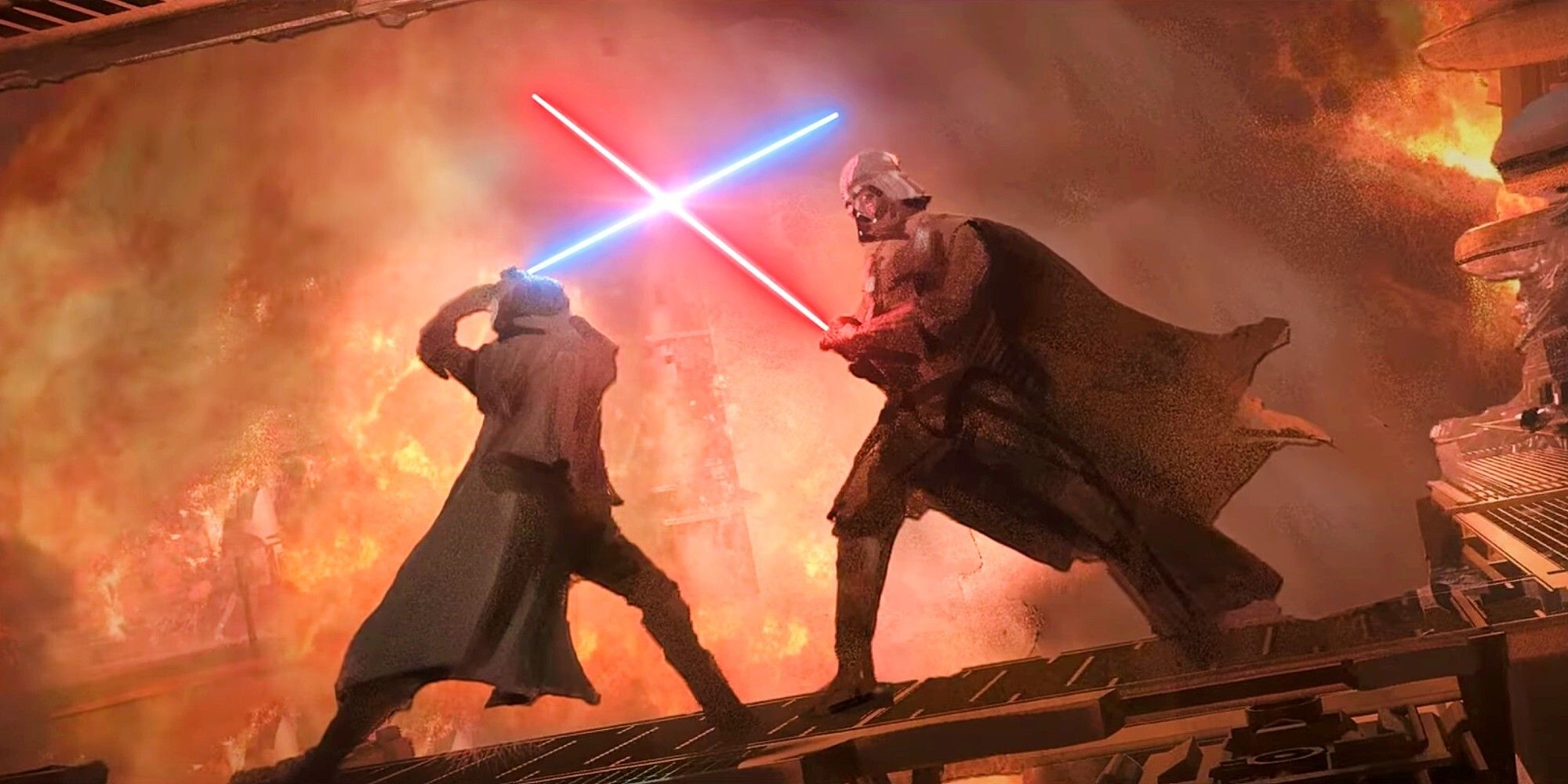The image is a highly detailed and dramatic digital art scene from Star Wars, capturing an intense lightsaber duel between Darth Vader and Luke Skywalker. Vader, wielding his iconic red lightsaber, advances from the right side of the frame toward Luke, who stands heroically on the left with his blue lightsaber. Their blades clash in an X formation, signifying a fierce battle. They are positioned on a metal grate or scaffolding, which appears to be tilted, adding dynamic tension to the scene. The background portrays a burning structure, possibly a temple or a city, engulfed in flames and smoke, providing a dramatic orange and red backdrop that accentuates the intensity of their confrontation. The landscape-oriented image emphasizes the fiery chaos surrounding them, making the focal point of their duel stand out even more.